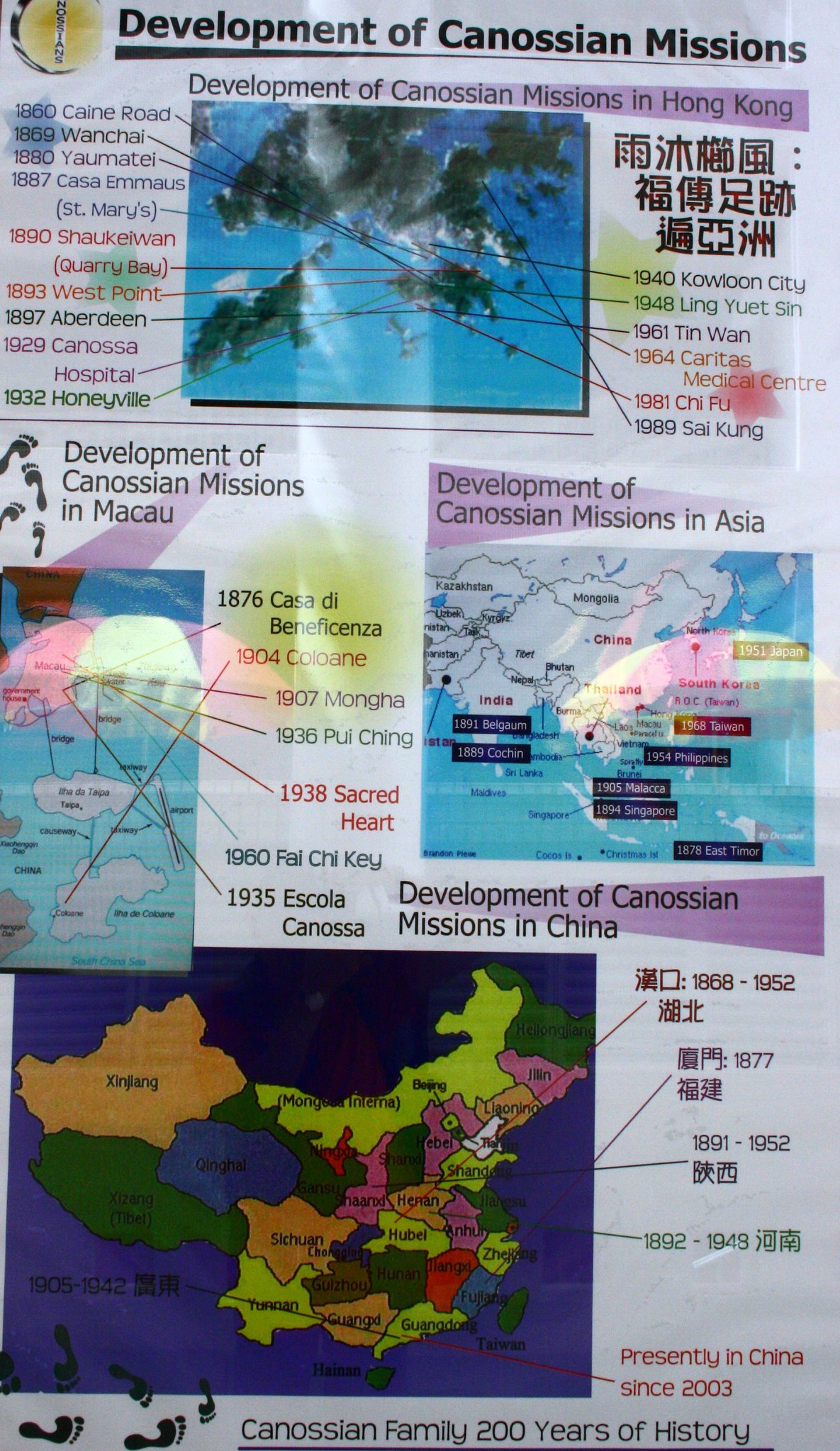The image displays a detailed poster titled "Development of Canossian Missions" prominently at the top. The main focus is on the Canossian Missions in specific Asian regions, particularly Hong Kong and Macau. The poster features three vibrant and colorful maps, specifically highlighting various locations within China, including Hong Kong, Macau, and other parts of Asia. The maps are adorned with a mix of English and Cantonese text, and various dates and locations are marked, such as "1860 Cane Road," "1869 Wan Chai," "1940 Kowloon City," and "1948 Ling Yat Sin." These dates likely denote significant events or the establishment of mission sites. The poster also underscores the historical development of these missions with tags like "Canossian Family: 200 Years of History." The timeline depicted spans notable years, suggesting the spread and evolution of the Canossian religious and humanitarian efforts throughout the region. The overall design is richly colorful, including a prominent use of purple behind some text, and features an icon of footprints, symbolizing the journey and impact of the Canossian Missions over the centuries.